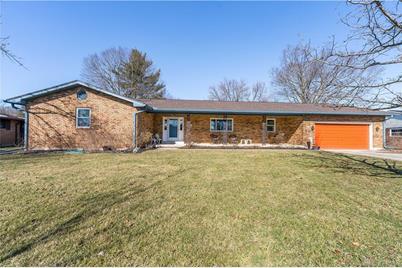This photograph captures an expansive outdoor scene featuring a one-story house against a backdrop of clear blue sky and trees. The house boasts a light brown, brick wall design and a prominent, triangular roof. It includes several small windows and a door, while to the right, an orange garage door with a shutter down is noticeable. In the foreground, a broad lawn covered in lush green grass stretches out, unmarred and spacious. Behind the house, a mix of trees can be seen, some with green leaves and others appearing dry. Sunlight bathes the entire scene, creating a warm and inviting atmosphere.